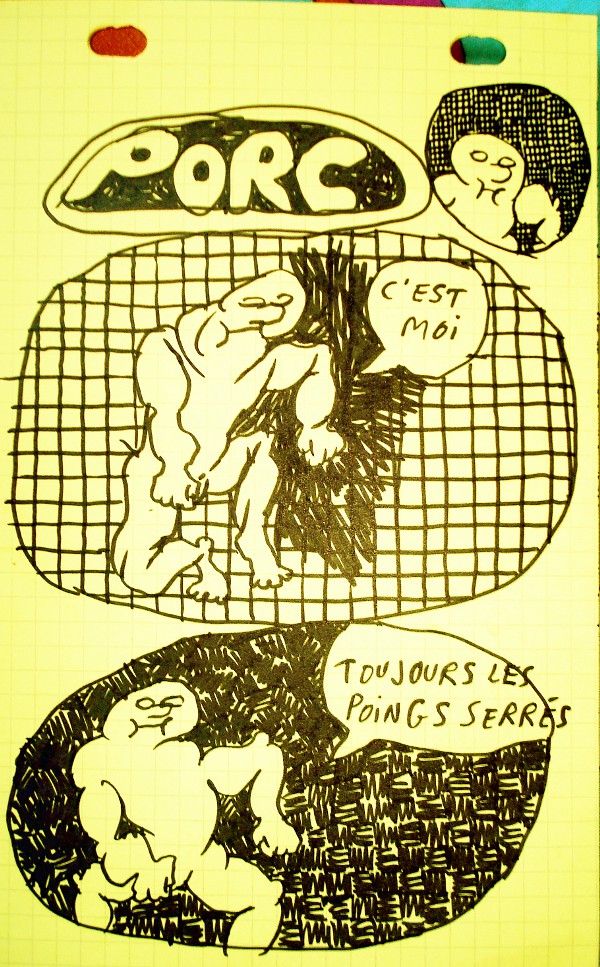The image is a detailed hand-drawn comic on yellow graph paper, held up by a red and green thumbtack with oval-shaped hole punches at the top. The title "P-O-R-C" is prominently displayed in bubble letters within a black oval at the top of the page. Next to the title, to the right, is a round black-filled panel featuring a peculiar character with hollow eyes and large cheeks. The comic consists of three circular panels: the uppermost panel bearing the solitary character, the middle panel showcasing a muscular version of the same character with the text "C'est Moi" beside it, and the bottom panel illustrating the same muscular figure with closed fists accompanied by the phrase "Toujours les Poinceres." The entire illustration exudes a whimsical, surreal quality with its black lettering and odd, monster-like figures, evoking a peculiar comic strip aesthetic.